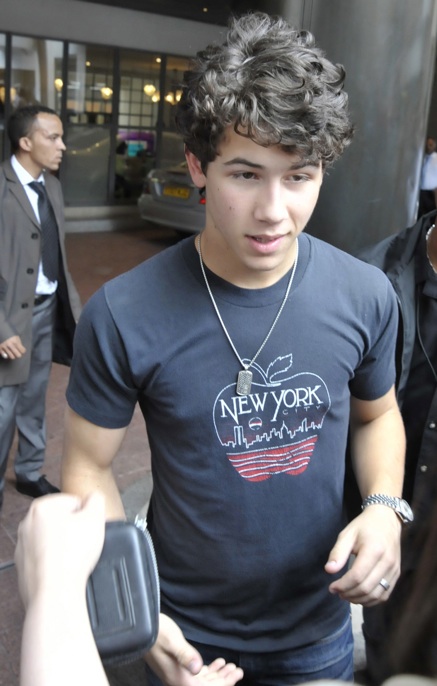The image depicts a young man with short black, curly-tipped hair and light skin, standing prominently in the center. He is wearing a dark navy t-shirt that features a graphic of an apple with "New York" written inside it and a hint of red at the apple’s base. He accessorizes with a silver necklace, which could be a dog tag, a wristwatch on his left wrist, and a wedding band on his ring finger. The setting appears to be outdoors, likely in the middle of the day, in front of a building with glass and columns, situated on brick flooring. Behind him, additional elements include a man in a gray trench coat with a tie and light blue pants, and other partial figures—an arm, a shoulder, and a face in the background. Scattered around are other individuals, and further back, buildings and cars can be seen. The color palette of the scene includes dark blue, tan, white, red, gray, and light blue, indicating a visually diverse backdrop.